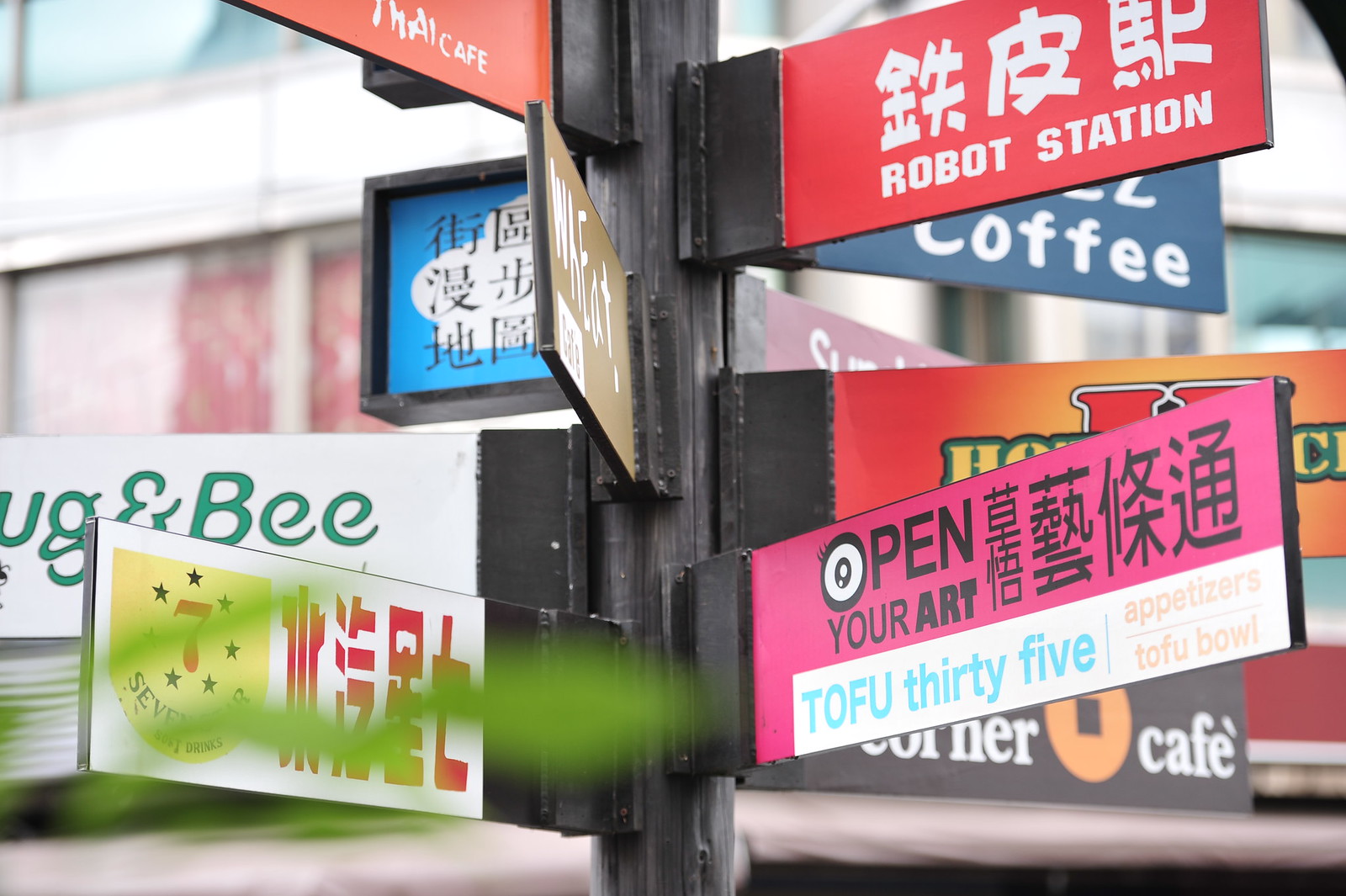This photograph depicts a bustling intersection adorned with approximately nine colorful and varied street signs affixed to a single post. At the top left, there is an orange sign for the "Thai Cafe." Directly below that is a blue sign with Asian characters that remain unreadable. To the upper right corner, a prominent red and white sign with both Asian characters and English text reads "Robot Station." Just behind Robot Station is another blue sign stating "Coffee" in white lettering.

Further down, there is a red sign partially obscured by a pink and white sign that reads "Open Your Art." Below this sign, a white insert with blue letters displays "Tofu 35," accompanied by a lighter font detailing "Appetizer's Tofu Bowl." Another distinct signage in red, yellow, and green appears to read "Can't Be Red," though it is partially blocked by other signs.

Additionally, there is a white sign with red Asian characters, partially hidden by greenery, and another sign labeled "Ugg & Bee" in green and white. A prominently black sign with white text reads "Corner Cafe." Intermingled within this visual array is another red and white sign that says "Seven" with seven stars and Asian writing, contributing to the dynamic and colorful atmosphere of the intersection.